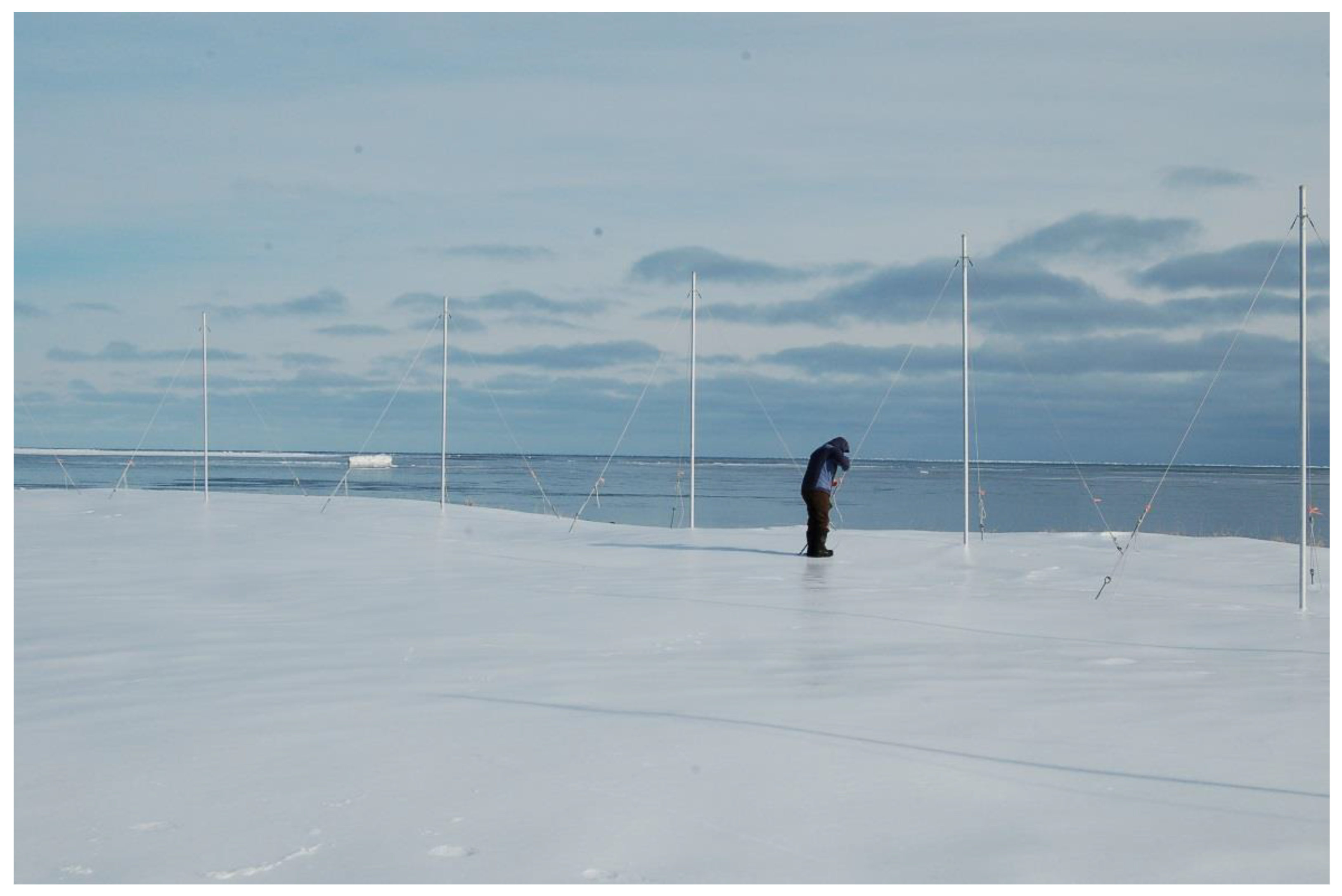In this slightly wider-than-tall image, we observe a snowy, frozen landscape featuring a flat expanse of ice reminiscent of an Arctic or Antarctic environment. The foreground showcases a tall, semi-transparent fence—possibly chain link—held upright by an array of poles and guy wires positioned across the scene. This fence, separating the icy expanse from a stretch of open water, extends laterally across the image.

A man dressed in a black snowsuit and black boots stands near the fence, appearing to adjust or tighten the wires. Shrouded in shadow, his specific features are indiscernible. The backdrop comprises a vast body of water, likely an ocean, that stretches into the distance.

The sky above occupies about half of the image, filled with a mix of lateral, dark clouds and wispy formations higher up, hinting at a cloudy, perhaps stormy day. A boat is faintly visible on the left-hand side of the water, further emphasizing the remote and frigid setting of this icy, meticulous scene.